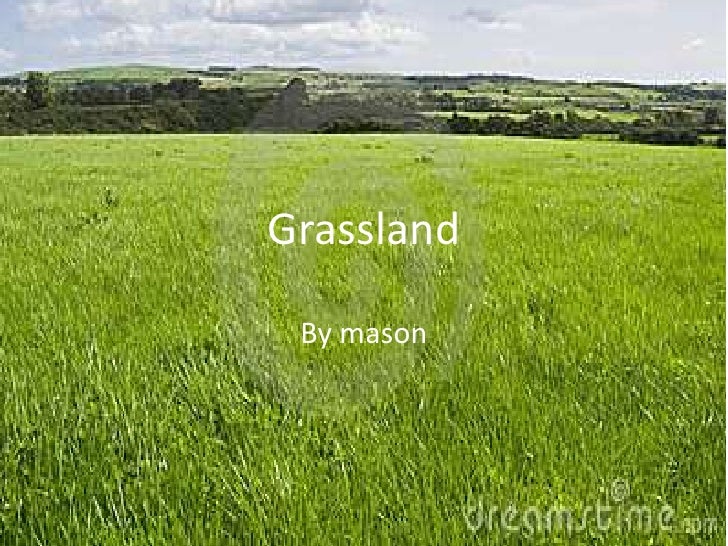The image showcases an expansive outdoor grassland, dominating the lower three-fourths to four-fifths of the frame with lush green and slightly yellow patches of grass, suggestive of sunlight. The midground features darker green shrubbery and trees, adding depth to the scene. In the furthest background, a hilltop with mixed grassy and wooded areas stretches along the horizon, adorned with some indistinct, elongated white buildings. Above the horizon, the pale blue sky is dotted with gray-white clouds. The entire composition is blurred, with clarity decreasing towards the background. White text in the center reads "Grassland by Mason," with Mason's 'M' in lowercase. In the bottom right corner, white transparent text reads "D-R-E-N-M-S-T-I-M-E," next to "E-D-M" and an emblem resembling an "at" symbol or a 'C' within a circle, followed by ".com".